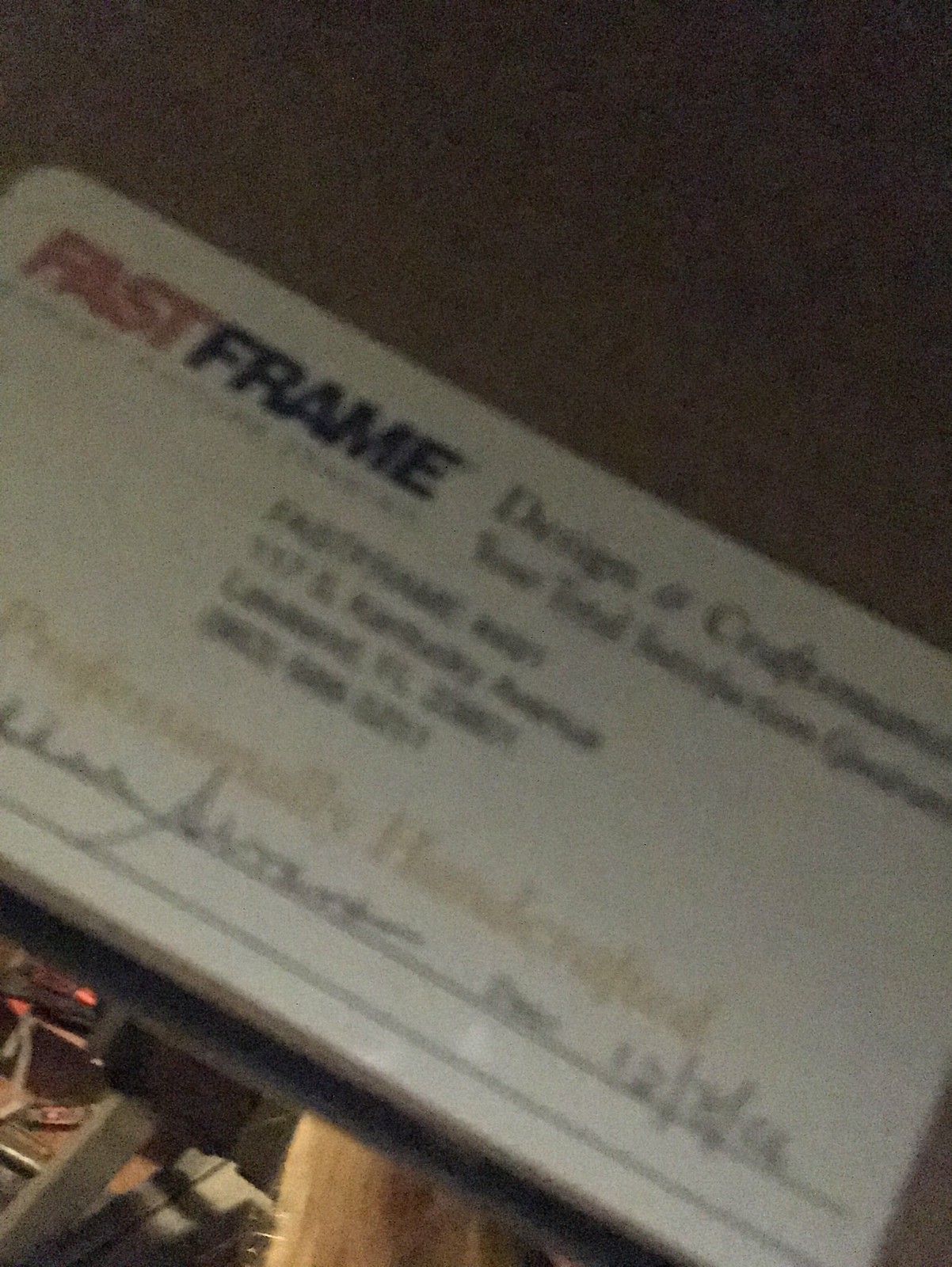The image depicts what appears to be a small, rectangular item, possibly a business card or a sticker affixed to the back of a photo frame. The item features a logo with the words "Fast Frame" prominently displayed in bold red and black text. The overall quality of the image is somewhat blurry, making it challenging to decipher all the details clearly. Below the logo, the text seems to read "Design," followed by another word that is likely "Craft," though the blurriness obscures it slightly.

At the center of the sticker, an address is printed, though the specifics are not entirely legible. The text appears to include the word "Handcrafted" in a gold-yellow hue, adding a touch of artisanal quality to the item.

Additionally, there is some handwriting on the item, featuring a date, though the exact numbers are difficult to discern. The background of the image hints at several objects, but their details are indistinct due to the poor clarity of the photo.

Overall, the item encapsulates elements of design and craftsmanship, possibly indicating a small business or artisan responsible for the framing or creation of the product to which the sticker is attached.